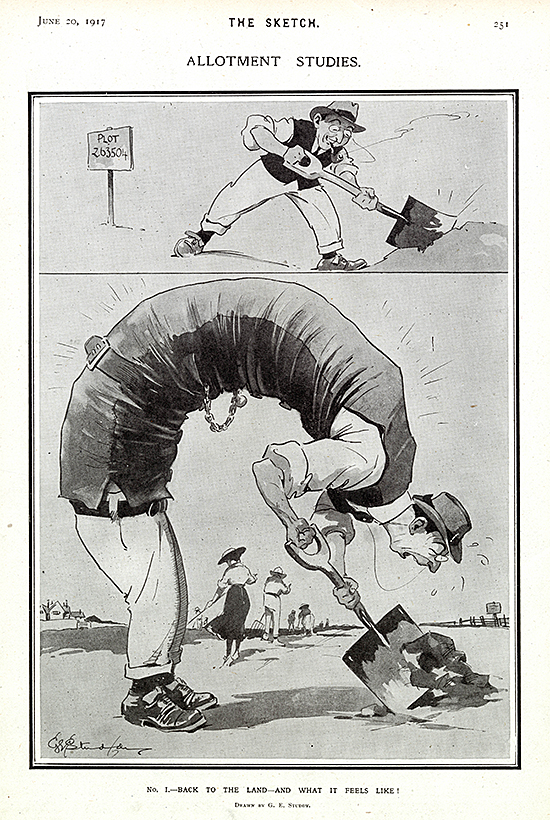This image is a page from a magazine, likely displaying a political cartoon. Set against a white background, the page is bordered by a black-outlined vertical rectangle containing two comic panels. At the top left of the image, the date "June 20th, 1917" is inscribed, while the top right corner features a small page number, likely "251." Centered between these elements is the title "The Sketch," under which another header reads "Allotment Studies."

The upper panel occupies roughly a third of the page and depicts a man wearing a hat, a black vest, white pants, and shoes, digging into a pile of dirt with a shovel. Behind him stands a sign labeled "Plot 263504."

The larger lower panel illustrates a surreal, elongated figure with an exceptionally long torso bent in a U-shape. This man, who could be the same individual from the top panel, also wields a shovel and appears to be digging, gazing at the ground in amazement. In the background, several other figures, possibly holding pitchforks or rakes, add depth to the scene. The bottom left corner of this panel includes an illegible signature, while the center bottom of the entire image features additional text reading "Number one, back to the land and what it feels like."

The image, rendered in black and white, is detailed and clear, vividly capturing the essence of early 20th-century satirical artwork.